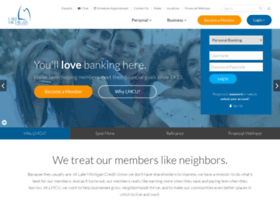The image is a screenshot of a webpage displayed on a desktop computer screen. The webpage features a large background picture of what appears to be a family of five. On the left side of the image stands a woman, next to her on the right is a man, and a boy with his hands resting on the man's shoulders. Adjacent to the boy is a little girl who is holding onto the shoulders of another woman. The overall color scheme of the webpage includes shades of blue, white, and orange. Although most of the text on the page is blurred and faint, a prominent text in dull grey and white reads "You'll love banking here." Below this text, there is an orange button and a transparent button with a white border.